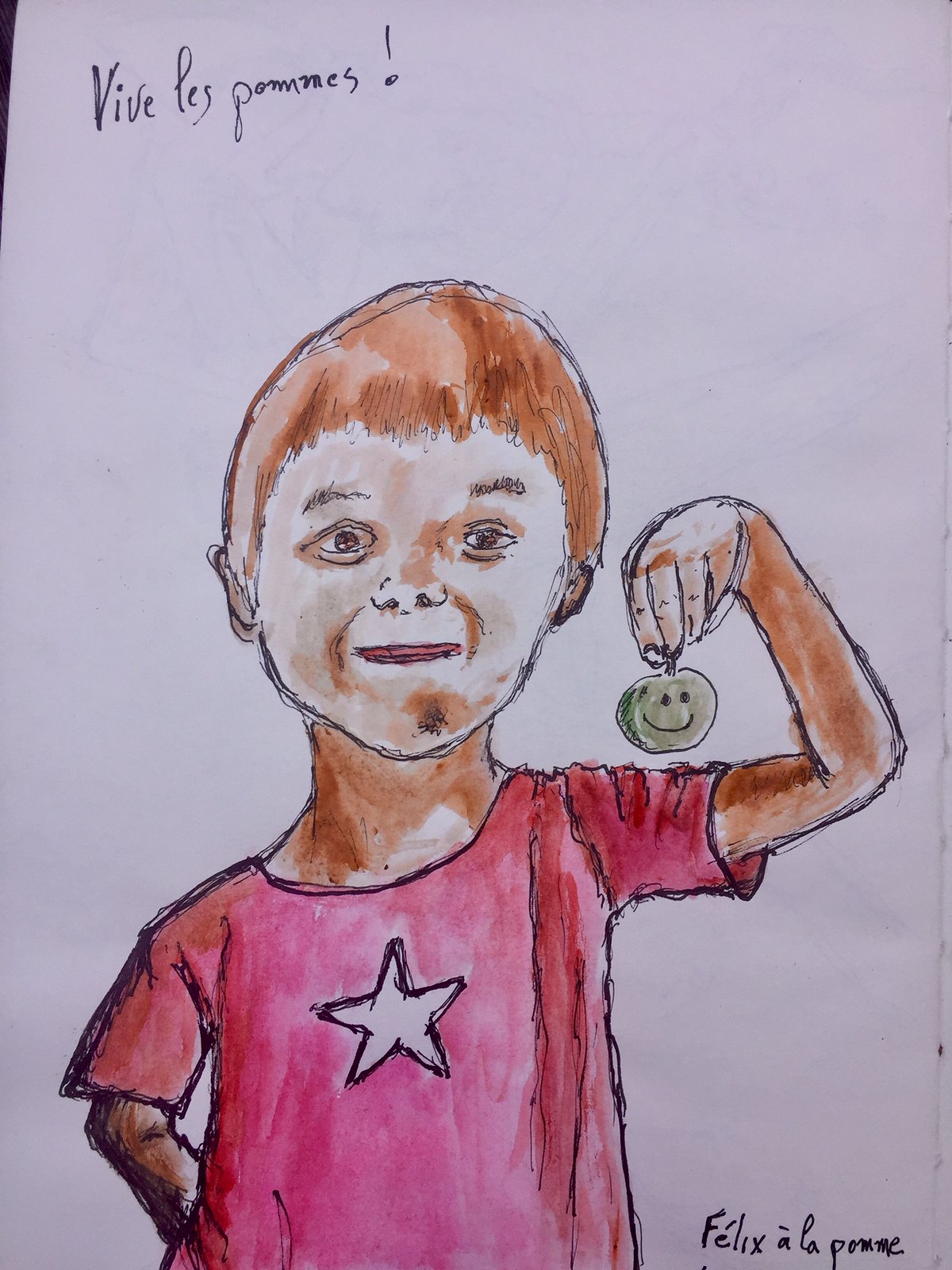A detailed drawing is displayed on white paper, depicting a young boy with reddish-brown hair. The boy's hair is short and somewhat tousled, with ears peeking out from beneath the strands on either side of his head. He has brownish eyes, dark eyebrows, and what appears to be a bit of dirt smudged on his face, giving him a playful, earthy look. The illustration, created with pen and possibly colored markers, features rough pencil lines beneath the ink.

In the boy's left hand, held close to his right cheek, is a green apple adorned with a cheerful smiley face. His right hand is concealed behind his back. He is wearing a vibrant red short-sleeved shirt, prominently decorated with a white star in the center of his chest.

In the top left corner of the drawing, the French phrase "Vive Les Pommes!" is written in bold letters, expressing an enthusiastic cheer for apples. In the bottom right corner, the signature "Felix L.A. Palme" is inscribed, indicating the artist's name.